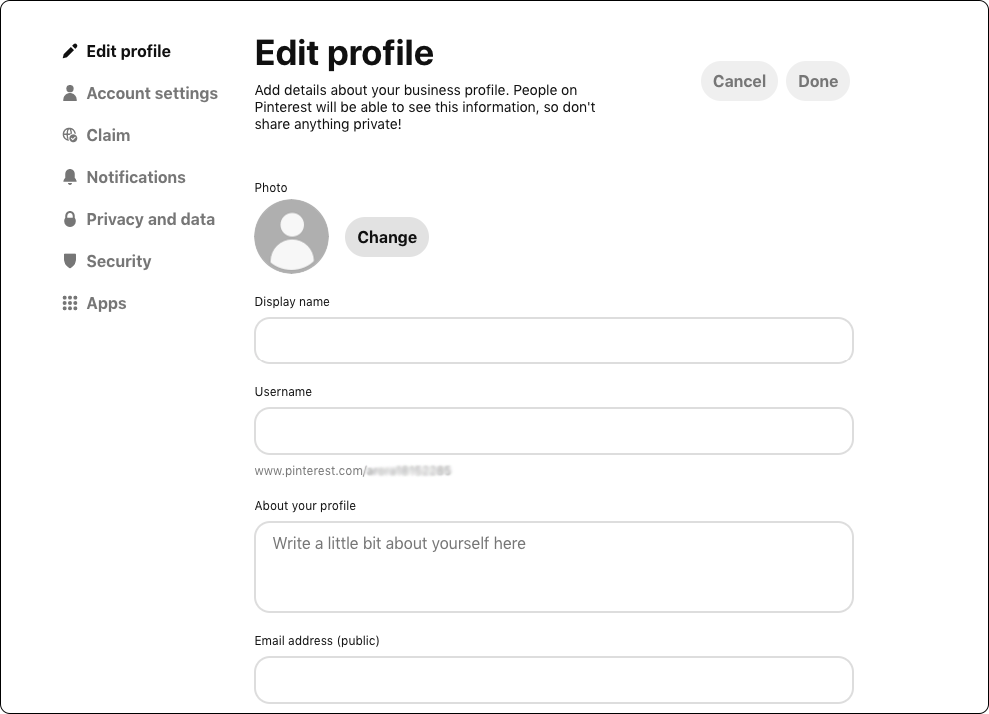This image is a landscape-mode screenshot of a profile edit form intended for business users on Pinterest. The form is organized into two columns. The left column features a white background, with the upper left-hand corner highlighting "Edit Profile" in bold text. Below that, a series of sections related to account management are listed: Account Settings, Claim, Notifications, Privacy and Data, Security, and Apps. Each of these sections is accompanied by its respective icon.

The main, more expansive right column is dedicated to the edit profile interface. At the top, an instructional message reads: "Add details about your business profile. People on Pinterest will be able to see this information, so don't share anything private." To the right of this message are two rounded, gray buttons labeled "Cancel" and "Done."

Beneath this, there is a placeholder for a photo, currently empty, accompanied by a gray "Change" button, which allows users to upload a new photo. The form itself consists of fields labeled "Display Name" and "Username," each requiring input from the user. Below the "Username" field, a partially obscured URL format is displayed as "www.pinterest.com/XXXX," where the specific user information is hidden for privacy reasons.

Further down, there is a section labeled "About Your Profile," encouraging users to write a brief description of their services for promotional purposes. Lastly, the form requests the user's public business email address, designated with the label "Email address public."

This screenshot visually and textually details the procedure for updating a Pinterest business profile, including sections for personal business information, a profile image, and social media linking.